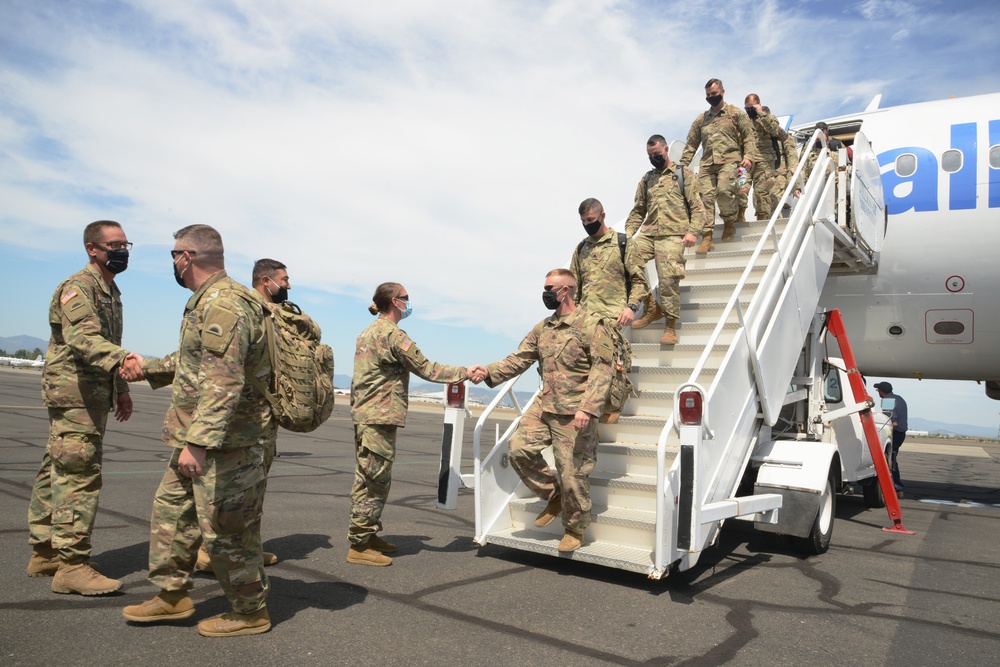The image depicts a group of military personnel in camouflage uniforms disembarking from a white airplane, whose side is partially adorned with the blue letters "ALL," possibly indicating an airline or organization. The soldiers are descending a white staircase onto a runway that features visible cracks and tar patches. Each soldier carries a backpack, suggesting they are returning from a tour of duty. At the base of the staircase, three individuals—one woman and two men—greet the soldiers with handshakes. All parties, including those greeting and disembarking, are wearing masks, hinting that the scene takes place during the height of the COVID-19 pandemic. The overcast sky, with occasional patches of blue, serves as a backdrop, along with distant mountains, contributing to the setting's solemn yet hopeful atmosphere.